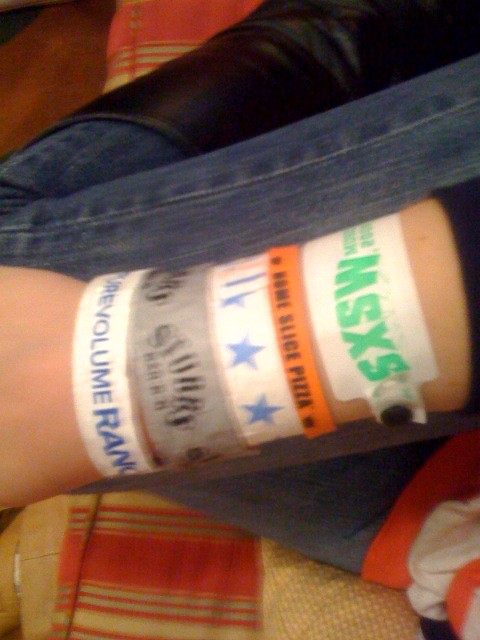The blurred, smartphone-taken photo features a woman's wrist adorned with multiple colorful bracelets, positioned in the center. Starting from top to bottom, the bracelets include a large white one with "MSXS" in green text, a small yellow one with "Sliced Pizza" in black text, a white one with blue stars, a gray one with unreadable black text, and a white one with blue text that reads "re-volume" or "RAM". The person, in blue jeans and knee-high black boots, is sitting on a seemingly beige couch covered with a red and gold striped blanket, alongside a golden and pink sheet and a white piece of fabric with orange stripes. Their forearm rests atop the blanket, partially revealing a dark brown floor at the photo's top left.